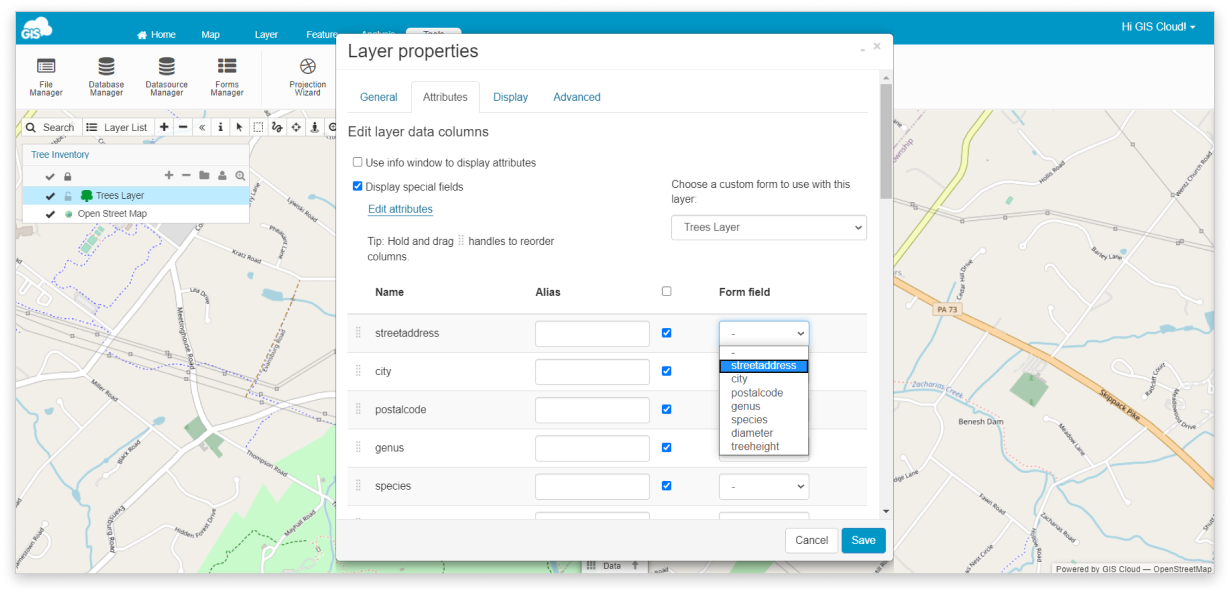Certainly! Here is a cleaned-up and detailed caption for the described image:

---

The image captures a GIS (Geographic Information System) user interface with a notable blue bar at the top. The bar features a cloud icon containing the letters "GIS" and includes various navigation buttons such as 'Home', 'Map', 'Layer', and 'Feature'. Directly beneath the blue bar is a toolbar with options like 'File Manager', 'Database Manager', 'Data Source Manager', 'Forms Manager', and 'Protection Wizard'. 

Further down, the interface displays a search bar along with a 'Layer List' section, which includes icons for adding layers ('plus'), removing layers ('minus'), navigating ('back arrow'), and accessing more information ('information icon'). The visible layers in the list are labeled as 'Tree Inventory' with sub-layers 'Lock' and 'Trees Layer', alongside a 'OpenStreetMap' layer.

The background, partly obscured by a pop-up window, reveals an underlying street map. The pop-up is labeled 'Layer Properties' and is segmented into several tabs: 'General Attributes', 'Display & Advanced', and 'Edit Layer Data Columns'. The 'General Attributes' section is shown with an option to 'Use info window to display attributes' and includes a marked checkbox for 'Display special fields'. A tip within the pop-up advises users to "Hold and drag handles to reorder columns".

Below the tip, a list of data columns is visible, which include 'Street Address', 'City', 'Postal Code', 'Genus', and 'Species'. The pop-up window is designed for editing and managing the properties of the selected map layer, allowing detailed customization of data representation.

---